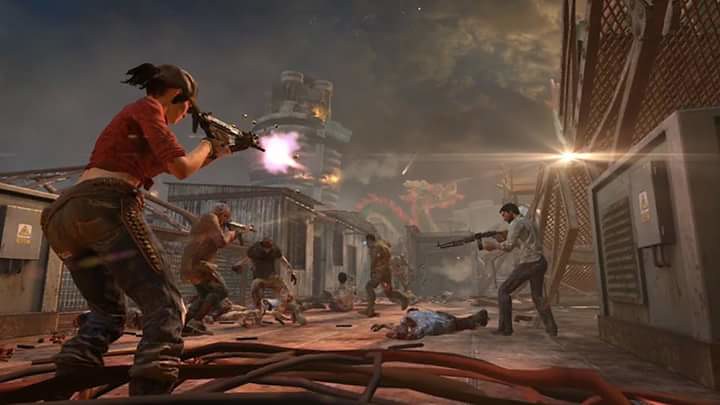In this dynamic and intense computer game graphic, the scene is set against a dark gray, cloudy sky, suggesting a high-stakes battle environment possibly atop a building or within a warehouse-like complex. Amidst the smoke and chaos of gunfire, a pivotal moment unfolds: a white woman with black hair partially visible from under her green hat is fervently firing her gun, a bright muzzle flash illuminating the barrel. She stands poised in a red shirt, dark pants, and boots with ammunition strapped to her leg, aiming her weapon at a man who appears to be in immediate danger. To her right, a grotesque zombie-like character adds a touch of horror to the fray. The foreground reveals a man in a blue shirt and brown pants, laying motionless on the ground—another casualty of this brutal firefight. Other combatants, including a man in a white shirt holding a gun, engage in the battle, standing over more fallen bodies. The scene is further detailed with small white buildings and large metal structures on either side, under a dim overhead light, all contributing to the gripping atmosphere of this digital conflict.